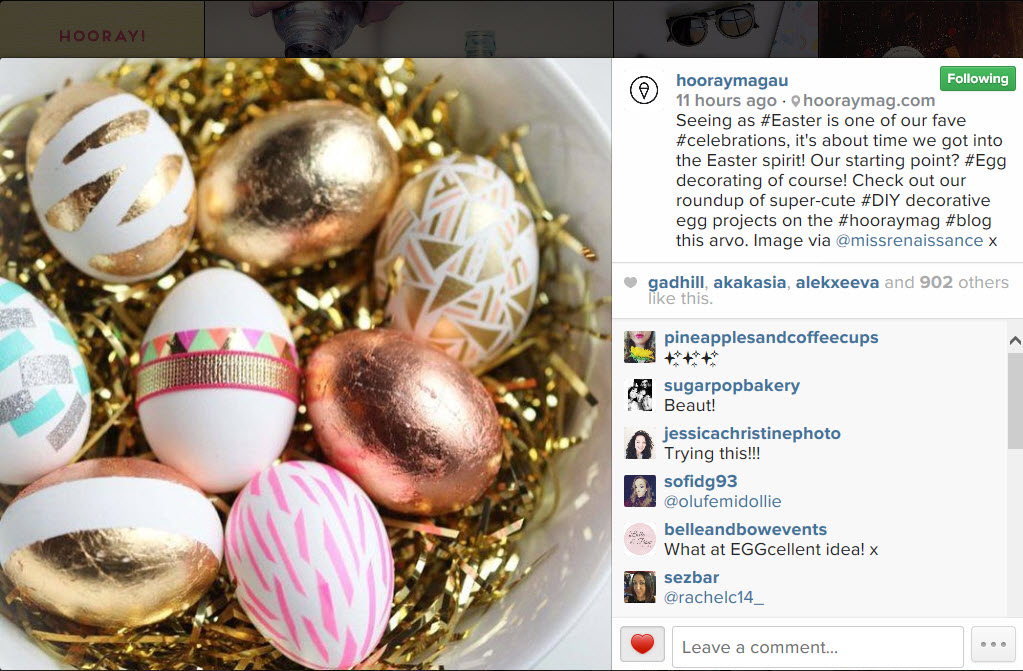The image features a festive Easter display, presented in remarkable detail. On the left side, shiny gold foil serves as a substitute for traditional Easter grass, creating a luxuriant nest. Nestled within the foil are an assortment of intricately decorated eggs, each unique in design. Among the collection, one can spot gold eggs adorned with delicate white lines, and shimmering golden pink eggs, reminiscent of rose gold. A pristine white egg is embellished with elegant pink lines, while another white egg boasts a central golden banner with a string of pink, green, white, and orange triangles above it. Another egg, positioned to the left, features a white base accented with silver and blue hues. The final egg in the array combines gold, pink, and white colors in a harmonious blend.

On the right side of the image, the text "Hooray M-A-G-A-U" can be seen at the top. The caption emphasizes the joy of Easter, stating, "Seeing as hashtag Easter is one of our fave celebrations, it's about time we got into the Easter spirit, our starting point, egg decorating of course. Check out the roundup of super cute hashtag DIY decorative egg projects on the blog." Below the image, comments from users with screen names in blue add a personal touch: Sugar Pot Bakery exclaims "Beaut," Jessica Christine Photo states "Trying this," and Bell and Bow Events adds "What an egg-cellent idea."